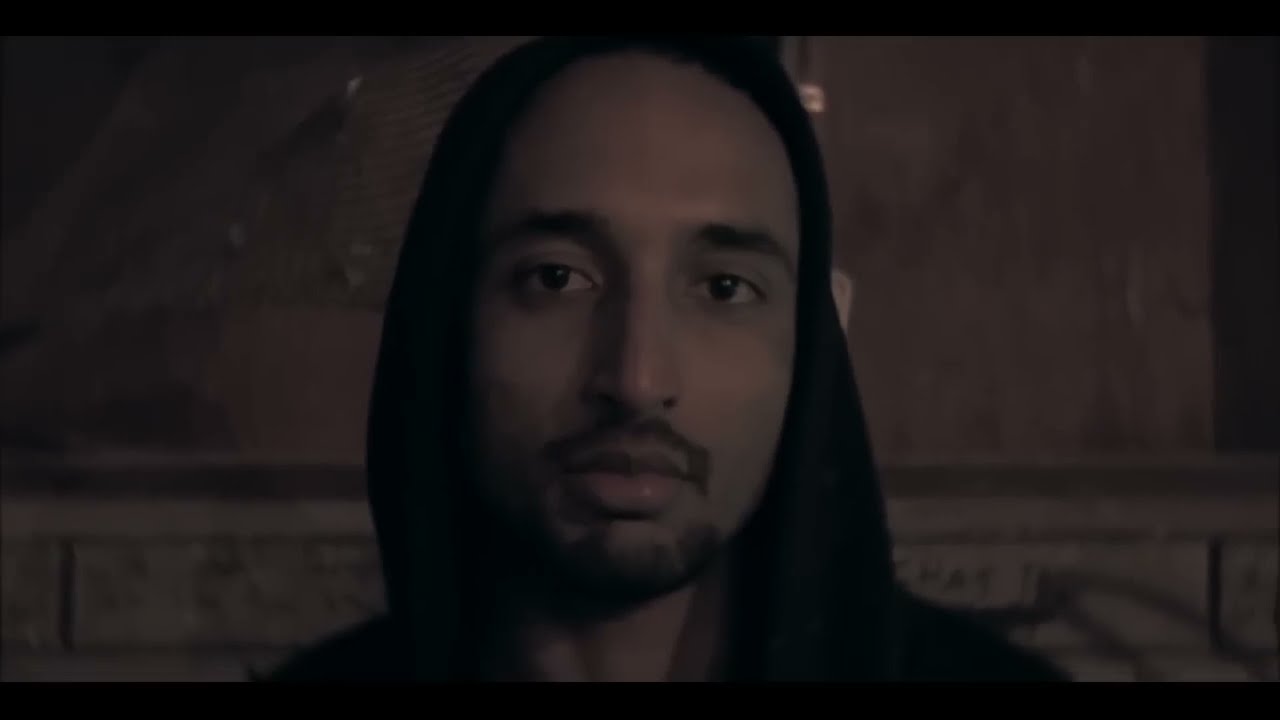In this color photograph, a Black man is positioned slightly to the right, appearing to be in mid-speech with his mouth open as he looks directly at the viewer. He is dressed in a casual outfit comprising a black knit winter hat that covers his hair, a blue nylon zip-up jacket, and a black T-shirt featuring a prominent white skull icon with unreadable lettering above it. He also sports a black goatee. The setting seems to be a back alley, characterized by a tan or brown background wall with some black markings. Behind him to the right, there's an open structure resembling a dumpster with chains visible on its left side. To the lower left of the frame, there is a white box containing what looks like a microphone. The overall atmosphere suggests an urban, possibly gritty backdrop.